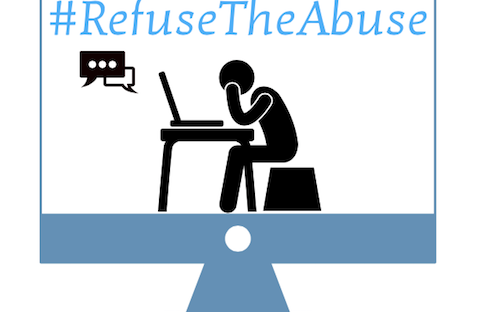The image resembles a blue MacBook monitor with a distinctive triangular base extending into a rectangular screen. At the top, in a stylized blue font, the hashtag “#RefuseTheAbuse” stands out against a white background. This text is somewhat distorted, with the "F" appearing incomplete. Below the hashtag, two symbols resembling a text conversation are depicted: one black speech bubble containing an ellipsis, and another white, empty speech bubble, both outlined in black. In the center of the image, a simple black silhouette of a person is seen sitting on a black block-like chair, hunched over a laptop on a desk. The figure's head is resting in their hand, indicating a gesture of distress or contemplation. The overall visual is framed within the borders of the MacBook-like monitor, which features a white button at the center below the screen, further highlighting the contrast of colors used in the image.